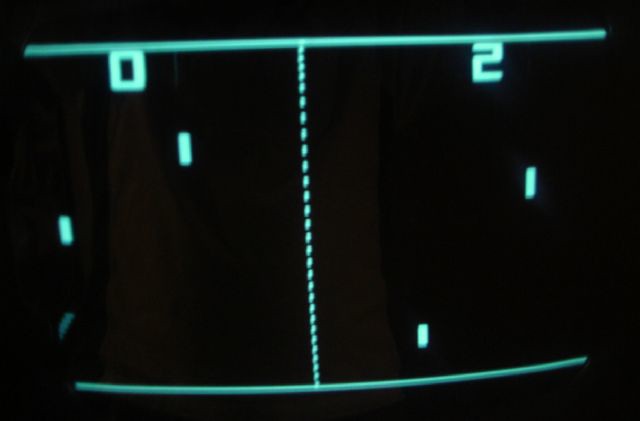A screenshot captures the classic arcade game Pong in action. On the screen, two thin green rectangles, situated on the left and right edges, serve as paddles for the players. These paddles are controlled to move vertically, up and down, within their respective boundaries. A small square ball bounces back and forth between the paddles, with each player striving to position their paddle just right to deflect the ball and score points. The minimalist design, characterized by simple geometric shapes and limited color palette, highlights the game's retro charm and enduring appeal.